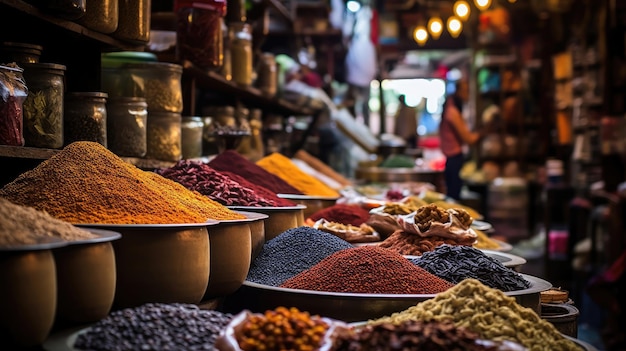This highly detailed and artistic photograph, likely generated by AI, captures the inside of a quaint, dimly lit spice shop. Prominently featured in the foreground is a long display table laden with large, copper-colored bowls and gray metal plates, each heaped with a variety of vibrant spices and herbs. The bowls, arranged primarily on the left, contain peaks of spices in hues of black, brown, green, yellow, and red, suggesting an array of textures from seeds to powders. Plates with similar mounds of spices are situated on the right side of the table, with some bowls and plates appearing seamlessly merged, characteristic of AI imagery. 

Behind this vivid display, a set of shelves on the left wall holds jars and cans likely filled with more spices for sale. The shop's lighting casts a warm, yellowish-brown glow, enhancing the dramatic ambiance while the background remains blurred, giving a sense of depth. Through the blur, daylight filters in from a distant doorway, hinting at people possibly milling about outside. This captivating scene evokes an atmosphere reminiscent of traditional spice markets found in places like Morocco or India.